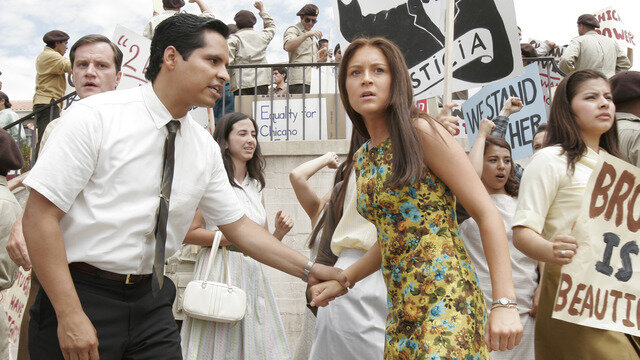The image portrays a scene from what appears to be a historical reenactment or a film set during a protest in the 1960s or 70s, advocating for Chicano rights. At the center of the photograph is a young, Hispanic couple. The man, muscular with short black hair and tan skin, wears a white short-sleeved dress shirt, a thin black tie, and black pants. He has his left arm around the wrist of a young woman, who wears a vibrant yellow dress adorned with blue, brown, and green floral patterns. She has long brown hair and a wristwatch.

The scene is bustling with energy, suggesting a large assembly or rally. Surrounding the couple are diverse individuals dressed in more subdued, pastel, or earth-toned colors, resembling church or Easter attire. Many participants in the background hold signs with messages like "Equality for Chicanos," "Brown is Beautiful," and "We Stand with Her." Among the crowd, some wear berets and sunglasses, adding to the charged atmosphere typical of a protest. The expressions on the couple’s faces convey a mix of shock and urgency; the man appears to be pleading with the woman, who looks scared and uncertain. This intense moment is set against a backdrop of about 15 to 20 people engaged in the fervent activities of the rally.